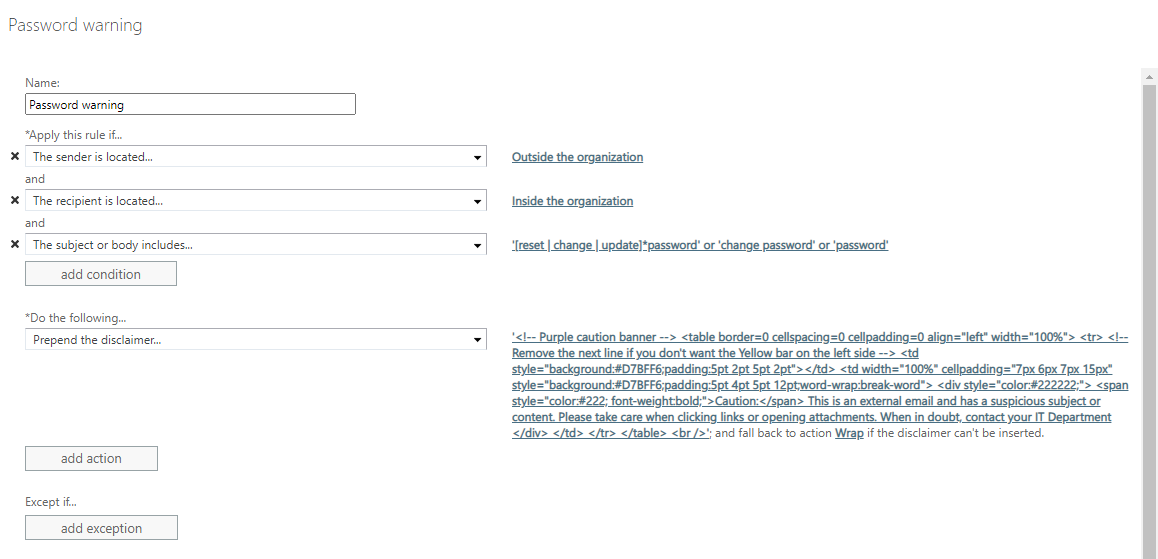The image displays a complex form with various written prompts and input fields. 

In the top left corner, in very faint writing, it says "Password Warning". Directly below that, "Name" is written, followed by a grey outlined box that also appears to say "Password Warning" with an asterisk. The text inside this box is too small to read clearly. 

On the left side of this form, there is an "X" icon, and beside it, a grey-outlined rectangle containing some words. To the right of this rectangle, there is an arrow pointing downward.

To the right of this section, the phrase "Outside this organization" is underlined, followed by "and". Below this is another "X" icon positioned next to another grey outlined box with text inside and a downward-pointing arrow on its right side.

The text "Inside the organization" is underlined in this section, followed by "and" and another "X" down below. There is yet another grey outlined box with words inside and a downward-pointing arrow. 

Further down is a light grey box with a darker grey outline stating "Add Condition". It is followed by "Do the following", a grey outlined box with words inside, and another downward-pointing arrow. 

Next to this, there is a paragraph that is partially underlined. On the left side of the form, there is another grey box outlined in darker grey which says "Add Action". Below that, it reads "Accept if", followed by a final grey rectangle outlined in darker grey with text inside.